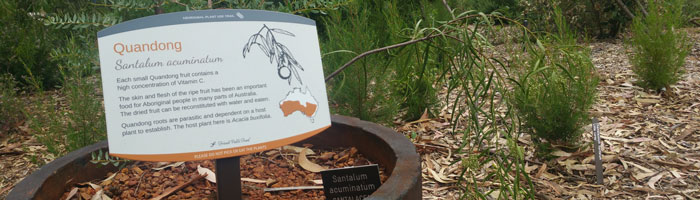This horizontal, rectangular outdoor image features a scene filled with earthy tones and greenery. The ground is covered in bark or dead leaves, creating a textured base that spans the entire frame. On the right, various shades of brown are interspersed with small green bushes, leading to a denser area of green vegetation, possibly trees or larger bushes, further in the background.

Dominating the left side of the image is a round pot filled with brown mulch. Within this pot stands a sign with a rectangular shape, curved at the top and bottom, and prominently labeled "Quandong" or "Kwandong" in orange letters. Below this title, the scientific name "Santalum acuminatum" is written in cursive. The sign includes a small black and white image of a plant, accompanied by a map in white and orange. Additionally, there are three small paragraphs of text beneath these elements, though the text is too tiny to read clearly. Surrounding this sign in the foreground is more mulch and green plants, seamlessly blending into the natural setting.